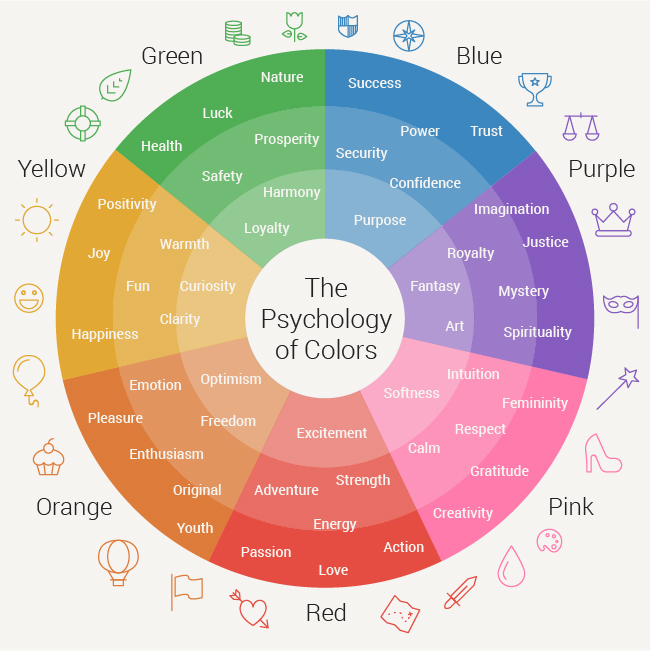The image showcases an infographic about the psychology of colors, set against a gray background. At the center, a beige circle contains the title "The Psychology of Colors" in black font. Around this central circle, the graphic is divided into multiple concentric rings, creating a colorful wheel segmented into seven sections, each representing a color of the rainbow. Starting from the bottom and moving clockwise, the colors are arranged as follows: red, orange, yellow, green, blue, purple, and pink.

Each color segment includes various descriptive words written in white font, detailing the psychological associations of that color. Red is linked to excitement, adventure, energy, and passion. Orange represents pleasure, enthusiasm, and optimism. Yellow connotes positivity. Green is associated with nature, health, luck, safety, prosperity, harmony, and loyalty. Blue stands for success, power, trust, security, and confidence. Purple symbolizes imagination, royalty, and possibly loyalty as per one description. Pink is related to femininity, respect, and creativity.

Scattered throughout the segments are small icons, such as a cupcake, a hot-air balloon, a teardrop, a shoe, and a crown, which visually reinforce the associated words. This detailed and colorful presentation aims to convey the complex and varied psychological impacts of different colors.